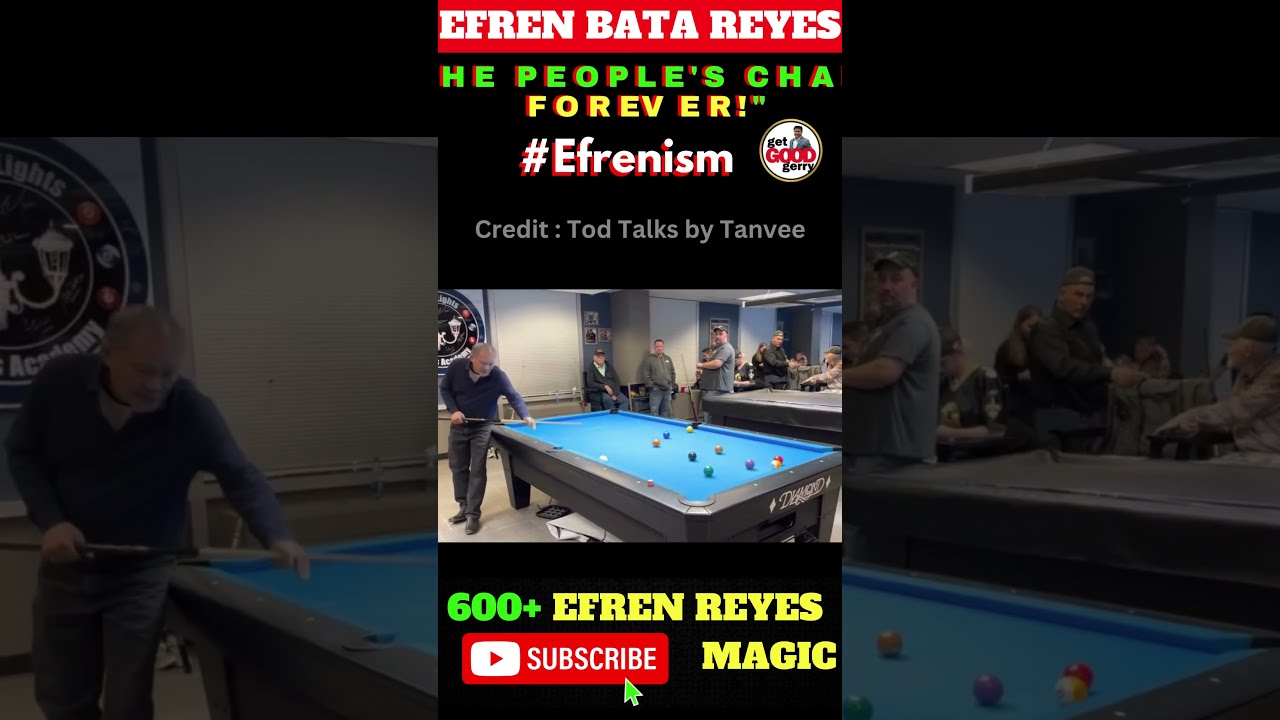The image is an advertisement primarily in a foreign language, prominently featuring renowned pool player Efren "Bata" Reyes. At the top of the image, in a small red banner with white capitalized letters, it says "EFREN BATA REYES." Below, in green letters, it reads "AT PEOPLE'S CHA" followed by the word "forever!" in yellow letters with an exclamation point and a double quotation mark. Further down, in white letters, there's the hashtag "#EFRENISM" and next to it a circular logo that says "Get Good Carry GERY." The credit for the ad, found in gray letters, reads "Credit: TOD talks by Tanvi."

The central portion of the image showcases a lively scene in a pool hall where a man dressed in a blue top and gray bottoms is about to make a shot on a blue-topped table branded with the word "Diamond." Behind him, four men and additional figures, including some women, can be seen either playing or observing the game. The pool table holds nine or ten balls arranged on its surface.

Below the image, green letters state "600+" and in yellow letters "EFREN REYES." Finally, in a red box with white letters, the word "subscribe" with an arrow is displayed. Adjacent to this, in yellow letters, is the word "magic."